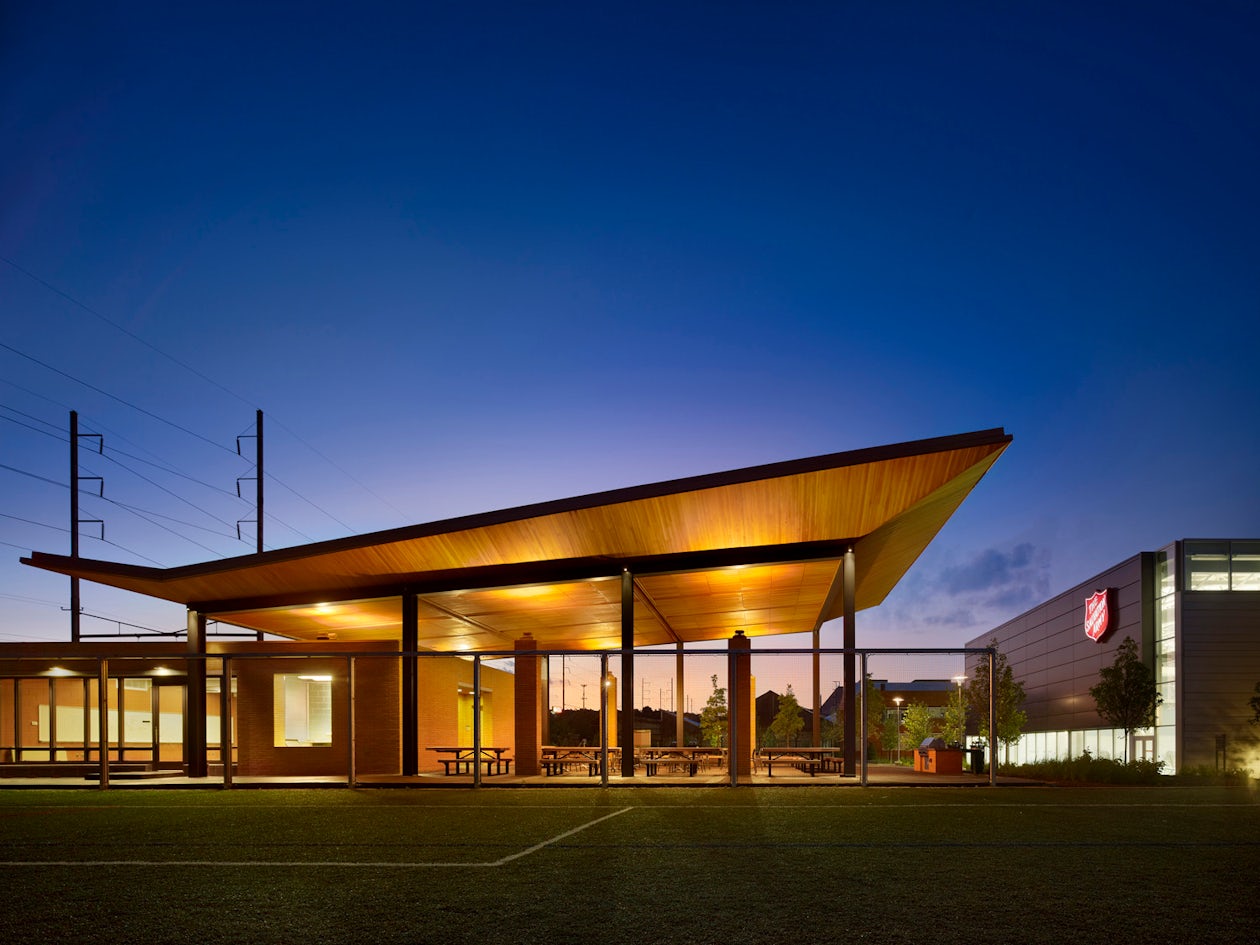The night sky is clear with just one cloud in the background, providing a serene backdrop to an urban scene. The image prominently features two buildings: the main structure is identified as a Salvation Army building, though its signage is barely visible unless zoomed in. Adjacent to this larger building is a smaller one, with a canopy-covered space bridging the gap between the two. The canopy shelters several benches, likely a designated area for breaks and quiet reflection. Power lines stretch across the picture, adding to the urban atmosphere. Overall, the composition captures a tranquil, yet structured night-time urban setting.